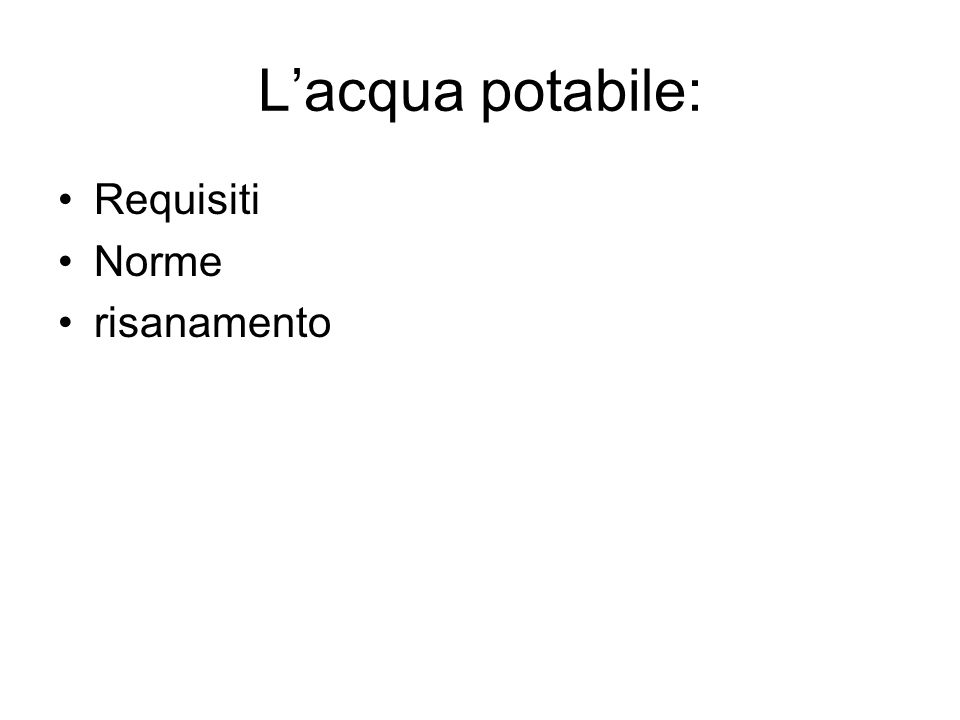The image features a simple layout with a predominantly white background. At the top, there is a large heading in Arial font which reads "L'Aqua Potable". This heading is significantly larger than the rest of the text and includes a colon at the end of the phrase. Below the heading, there are three bullet points with text in a non-English language. The first bullet point reads "Requisitee" with a capital 'R'. The second bullet point is "Norm" with a capital 'N', and the third bullet point is "resentimento," which is the only bullet point that starts with a lowercase letter 'r'. The design is straightforward and uncluttered, emphasizing the listed terms under the clear heading.